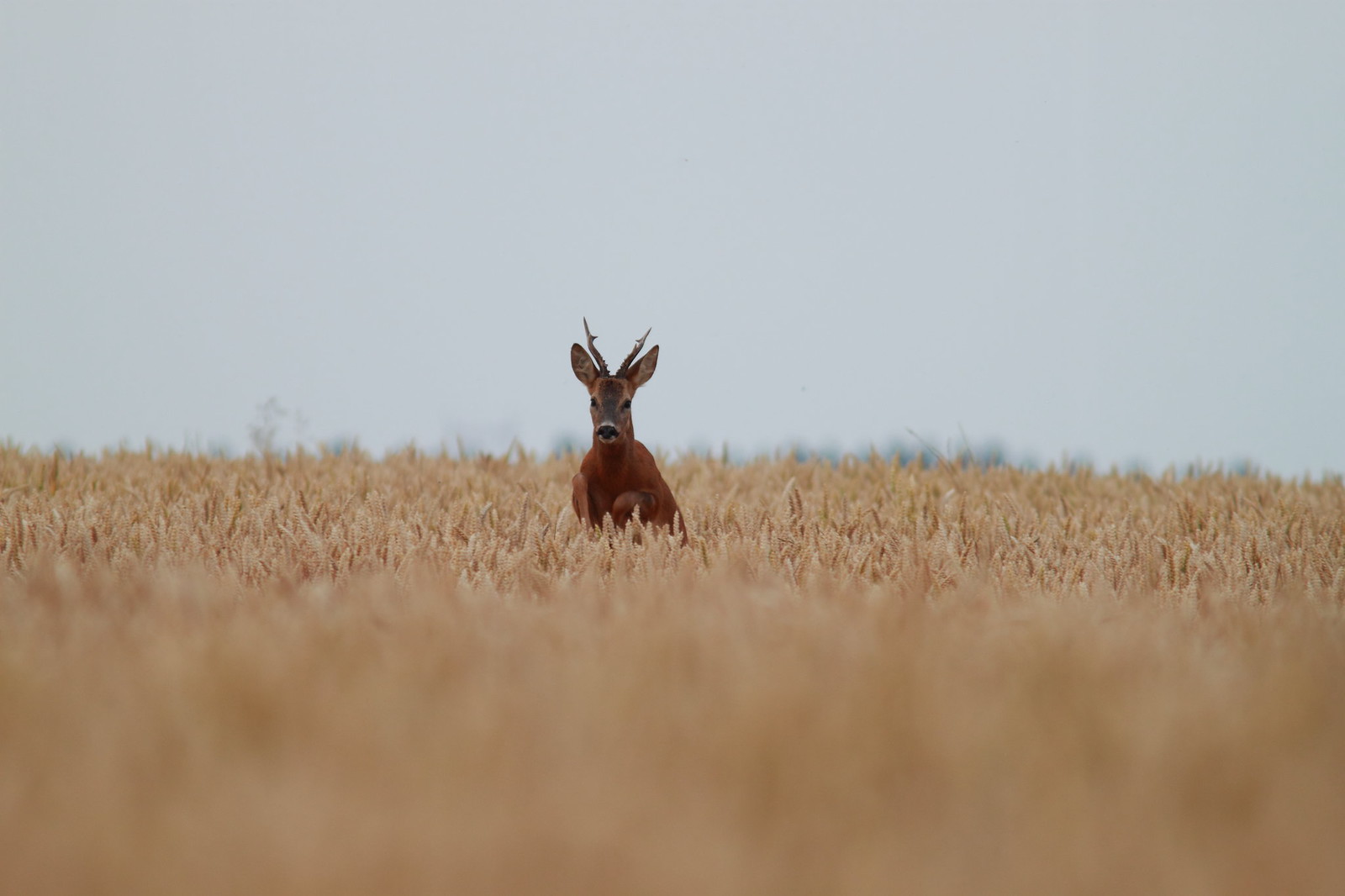The photograph captures a dynamic scene of a young buck in mid-stride, running directly towards the camera through a vast, light brown field of reeds or possibly wheat. Dominating the center of the image, the deer has short, developing antlers protruding above its pointed ears and a dark brownish-gray snout, contrasting against its solid medium brown body. With its front legs lifted, the deer appears poised, almost as if caught between strides. The lower portion of the image is a blur of light and medium brown hues, suggesting close-up grass or straw in the foreground, while the clear, bluish-gray sky stretches across the top, emphasizing the outdoor, daytime setting. The seamless blend of the blurred foreground and the sharp focus on the deer within the expansive field creates a sense of motion and immediacy, drawing the viewer's attention to the poised grace of the buck.